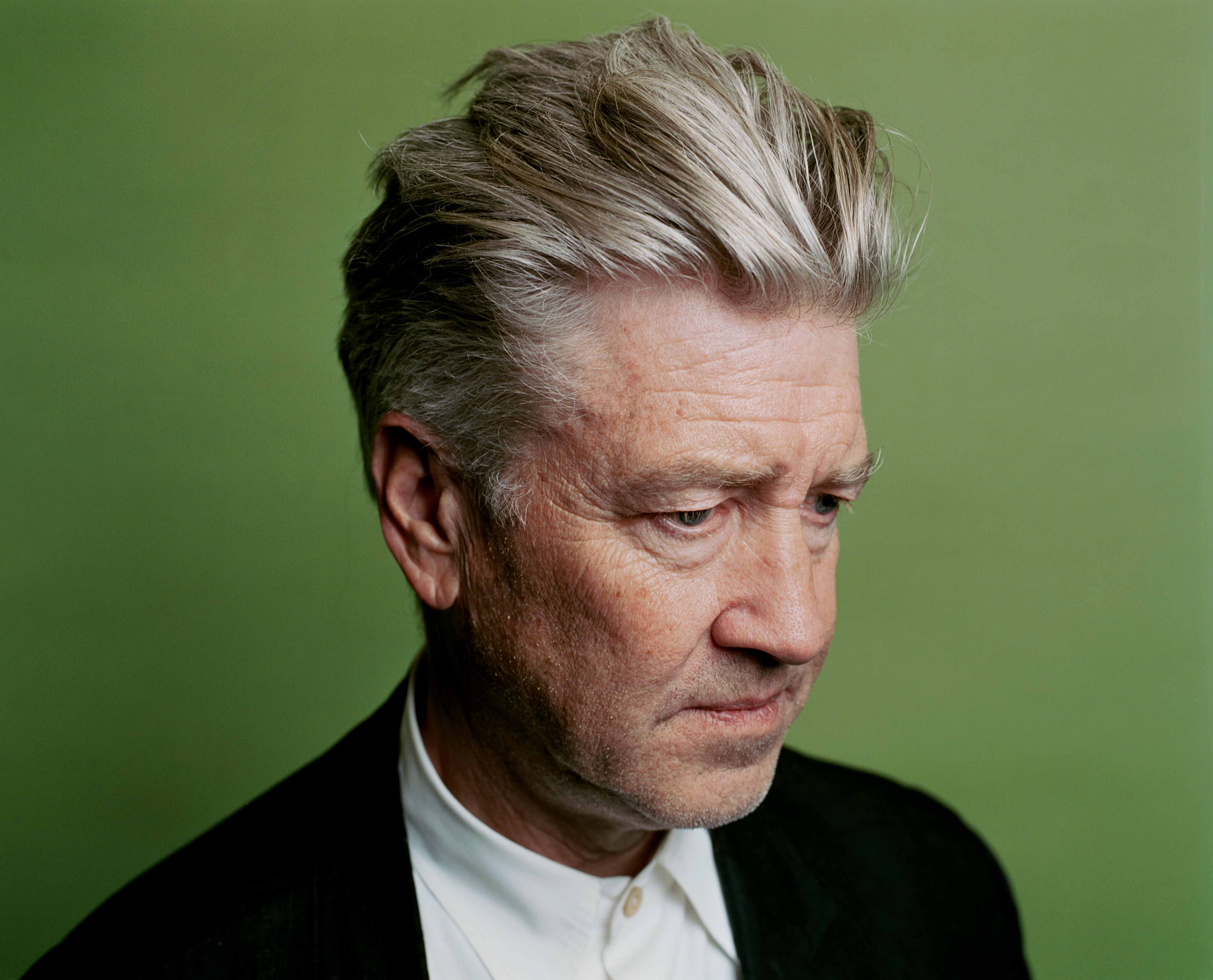The photograph is a close-up portrait of a man in his early to mid-60s, taken from his upper shoulders to the top of his head. He is dressed in a black coat over a white button-up collared shirt with tan buttons. He has light gray eyes and short gray hair that is swept backwards, with slightly longer strands on top. Despite the varied descriptions, his hair color appears to be a mix of gray and blonde, adding a faded, mature look. The man has some stubble on his cheeks, chin, and upper lip, showing a mix of white and black hairs.

His expression is contemplative as he looks towards the bottom right of the photograph. The background is a green color, possibly greenish-brown, with the lighting making the left side of the photograph significantly darker than the right. The man's face is somewhat overexposed in terms of lighting, but the area behind his right ear and his neck darkens considerably. The photograph's composition gives it a nearly perfect square shape, enhancing the formal and reflective mood of the portrait.